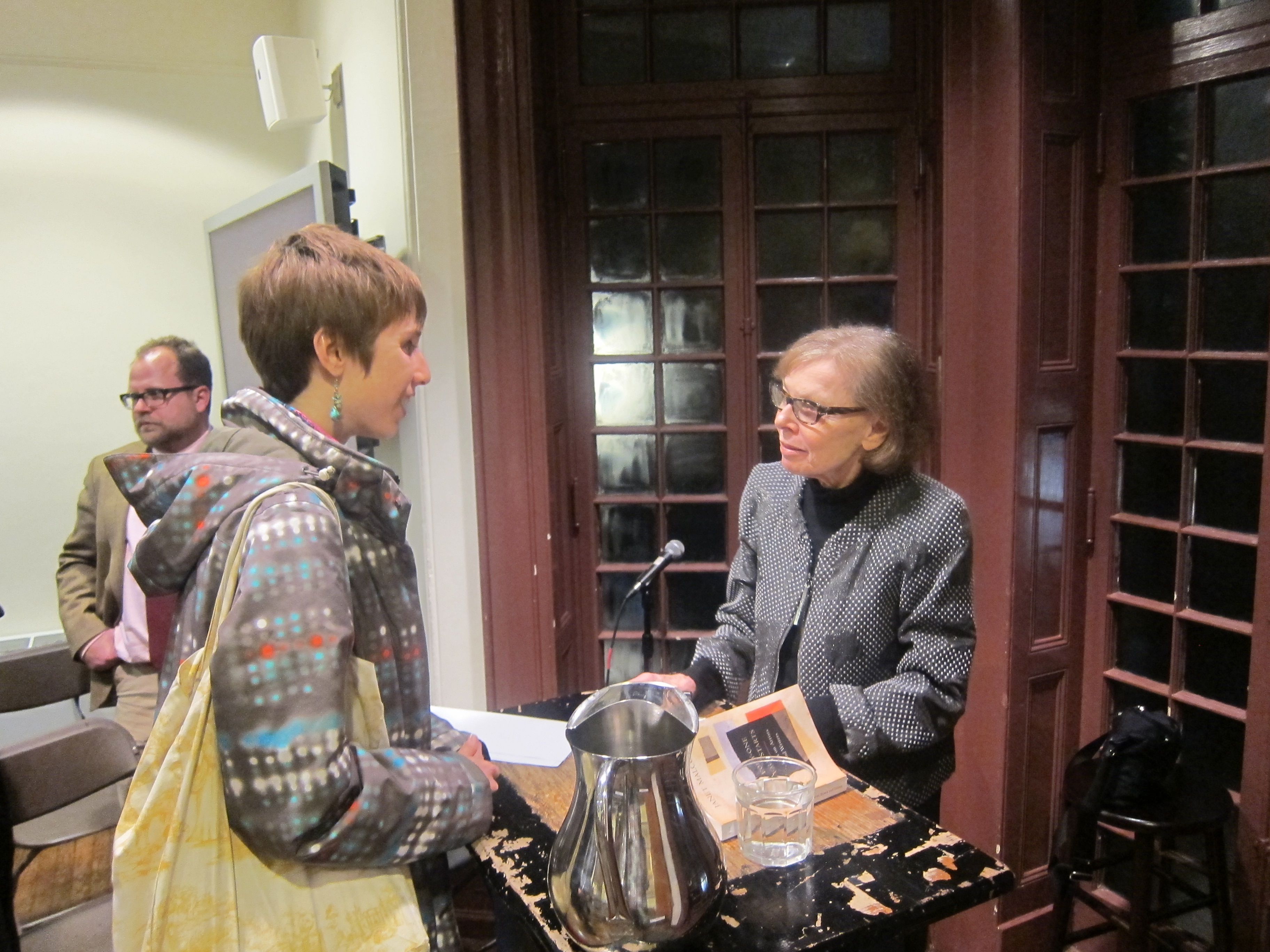The photograph captures a detailed scene of an indoor book signing event. Featured prominently on the right side of the image is an older woman, who appears to be an author in her late 60s or early 70s, seated behind a weathered, black podium that has noticeable dings and an attached microphone. She has on dark-rimmed glasses and is wearing a gray tweed jacket over a black shirt. On her right rests a small black stool and a black bag. 

Engaged in conversation with the older woman is a younger woman, likely in her early 20s, standing on the left side of the image. She has short reddish-brown hair styled in a pixie cut, is smiling, and carries a tan shoulder bag over her right shoulder. She is dressed in a gray jacket featuring a red, blue, and white pattern with a hood. The younger woman's right arm is bent at the elbow, as if she has placed a book on the podium, possibly for the older woman to sign. 

In the center foreground of the image, atop the podium, rests a silver water pitcher filled with ice water alongside a half-filled glass of water, suggesting refreshments for the event. 

Behind the two women are burgundy-colored, grid-style glass doors and windows, adding an ornate backdrop to the setting. Further into the background, near a corner of the room, stands a man possibly in his late 40s. He sports a highly recessed hairline with brown hair on the sides, dark-rimmed glasses, and is dressed in a tan sports jacket, light tan trousers, and a white shirt. The white walls and the detailed wood-framed window or door area in the background further frame the event scene, adding an air of elegance to the setting.